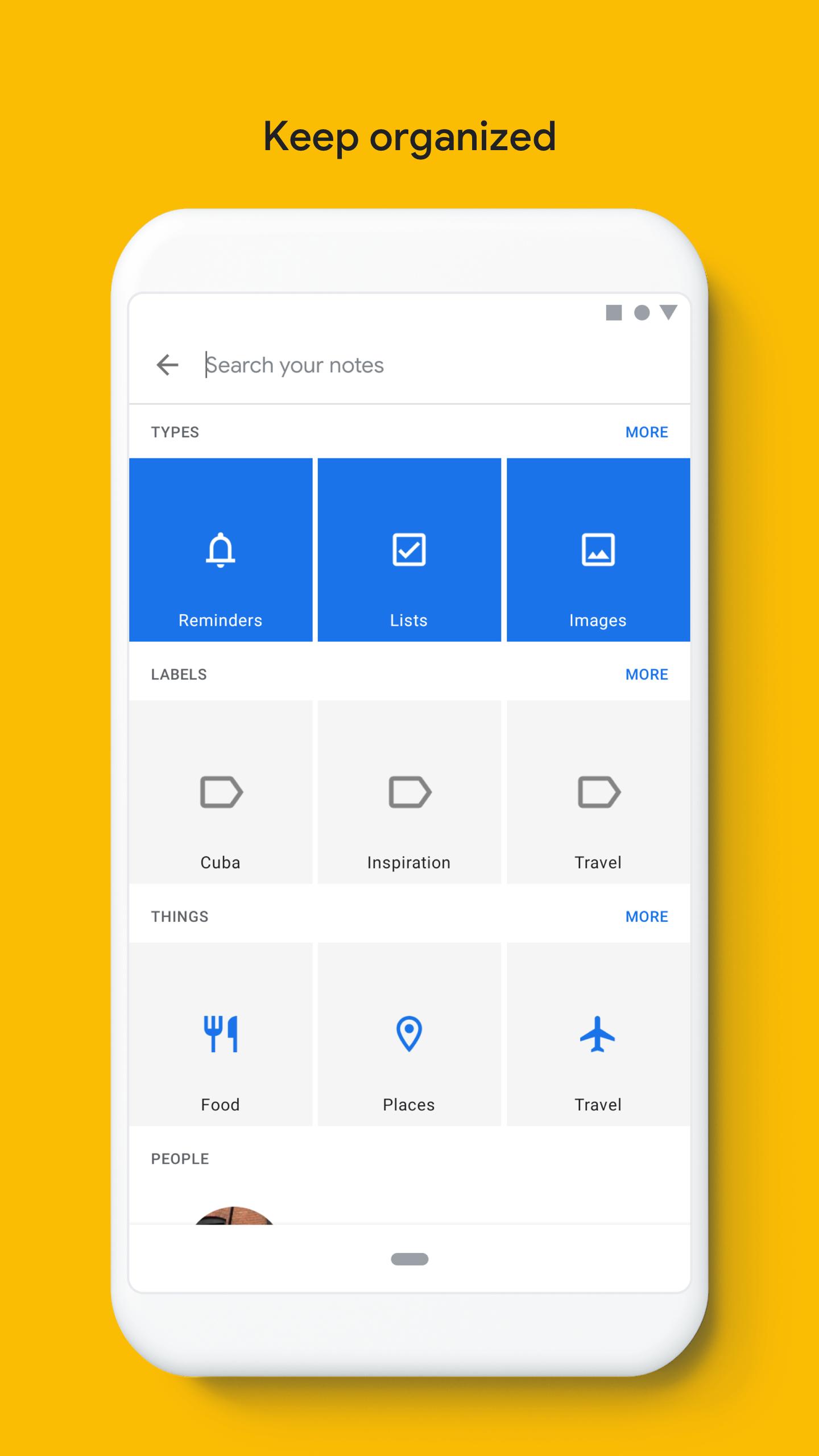The image features a mobile device placed on a vibrant yellowish-orange background. The color scheme of the device's interface includes yellow, blue, and white, reminiscent of Walmart’s brand colors. On the screen, black text on the orange section reads, "Keep organized." Following this, there is another prompt, "Search your notes on the device," though it appears to be left blank in this instance.

The interface is categorized into several sections:

1. **Type**: This section includes organizational options listed as "Reminders," "Lists," and "Images," with an additional link to "More."
   
2. **Labels**: Under this category, there are three labels: "Cuba," "Inspiration," and "Travel," along with an extra link to "More."
   
3. **Things**: This involves tags such as "Food," "Places," and "Travel," also with an option to "More."

At the lower part of the device’s screen, there’s a circular element containing a photograph, labeled "People." This section stands out against a slight purple tint in the background, providing contrast and drawing attention to the user’s content related to people.

Overall, the screen showcases an organized and visually appealing interface designed to help users manage their notes, reminders, and labels effectively.